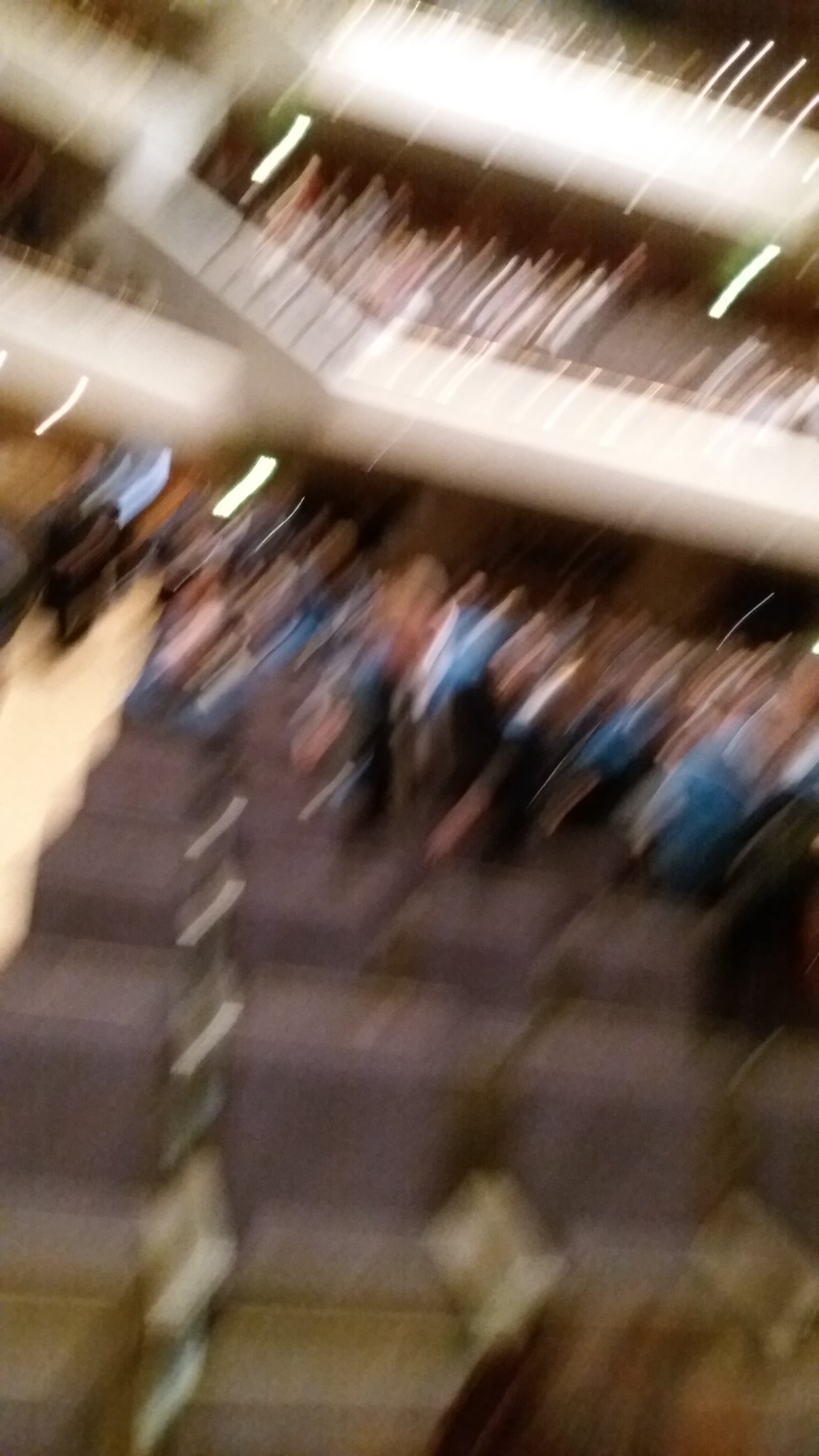A very blurry image captures a moment at a sporting stadium, possibly a football, soccer, or basketball arena. The photo, taken vertically on a cell phone, centers on the first and second rows of seats, which are notably empty. These seats are a striking royal purple, with three to four visible in each row. Beyond these vacant seats, a number of spectators can be seen. Some individuals are making their way up stairs located to the left side of the frame, heading away from the camera. Among the crowd, one person stands out as they are in the process of standing up and moving toward the aisle to their right, which is to the camera's left. The stadium features three tiers, each separated by white sections, adding a structured aesthetic to the scene. The overall blur lends an abstract quality to the otherwise vibrant and bustling atmosphere.